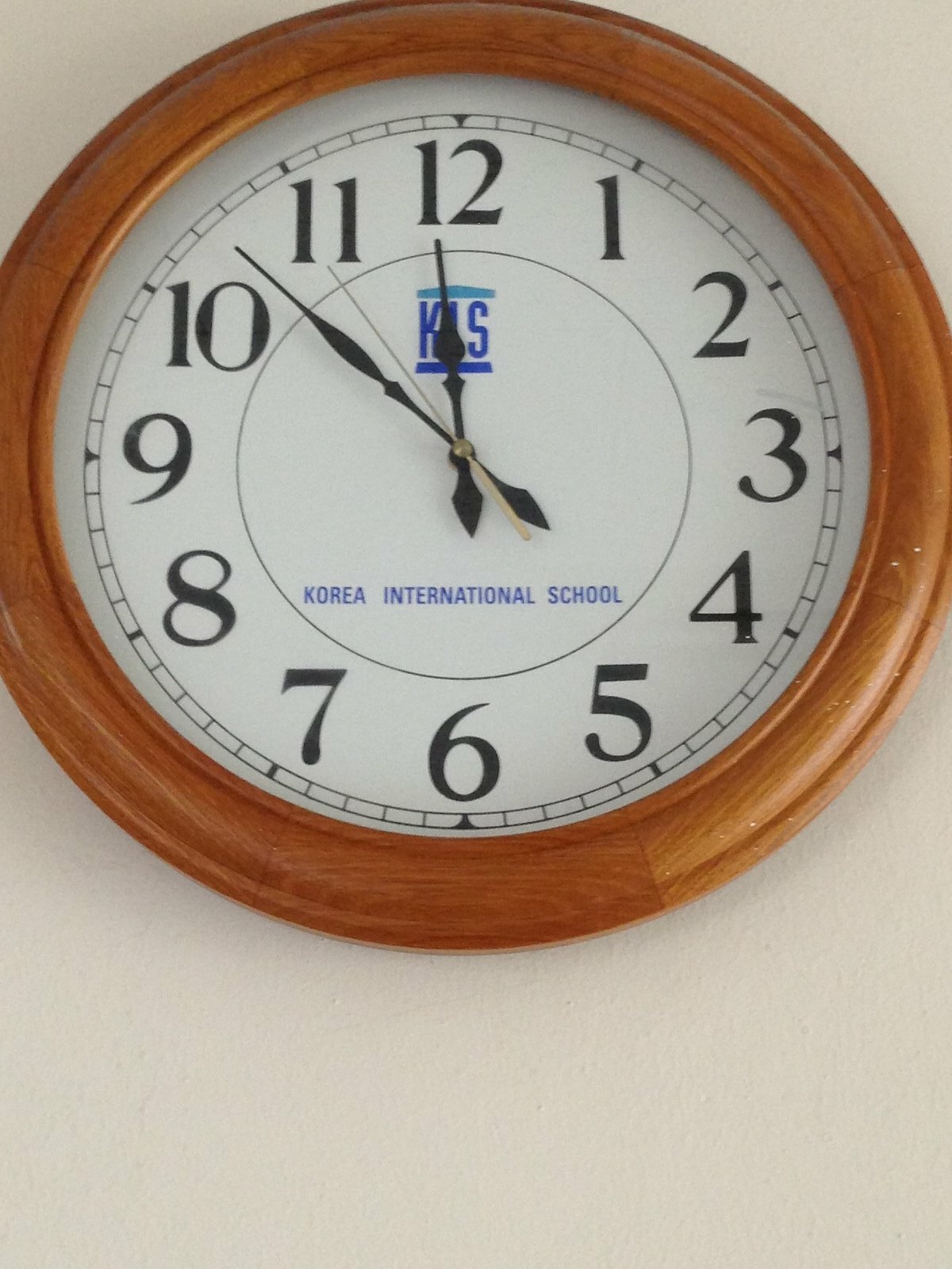This photograph features a detailed image of a circular analog wall clock with a prominent, decorative wooden frame that appears lathe-turned. The clock's face is white, providing a sharp contrast to the black numbers arranged in a traditional 1-12 sequence around its circumference. The hour and minute hands, both black and somewhat ornate with slight curves, stand out clearly against the white background. The second hand is thin and gold, adding a subtle, elegant touch.

In addition to the numbers, there are markings for each minute, with thicker lines demarcating the five-minute intervals, enhancing the clock's readability. Notably, the 3, 6, 9, and 12 o'clock positions feature triangular markers for further clarity. 

The clock also incorporates additional design elements: a smaller inner circle around the central point and a logo situated just under the 12, depicting the initials KIS with a house-shaped top in a gradient from light to dark blue. The text "Korea International School" appears in blue capital letters below the clock hands, positioned above the 6. These features collectively contribute to the clock's functional and aesthetic appeal.